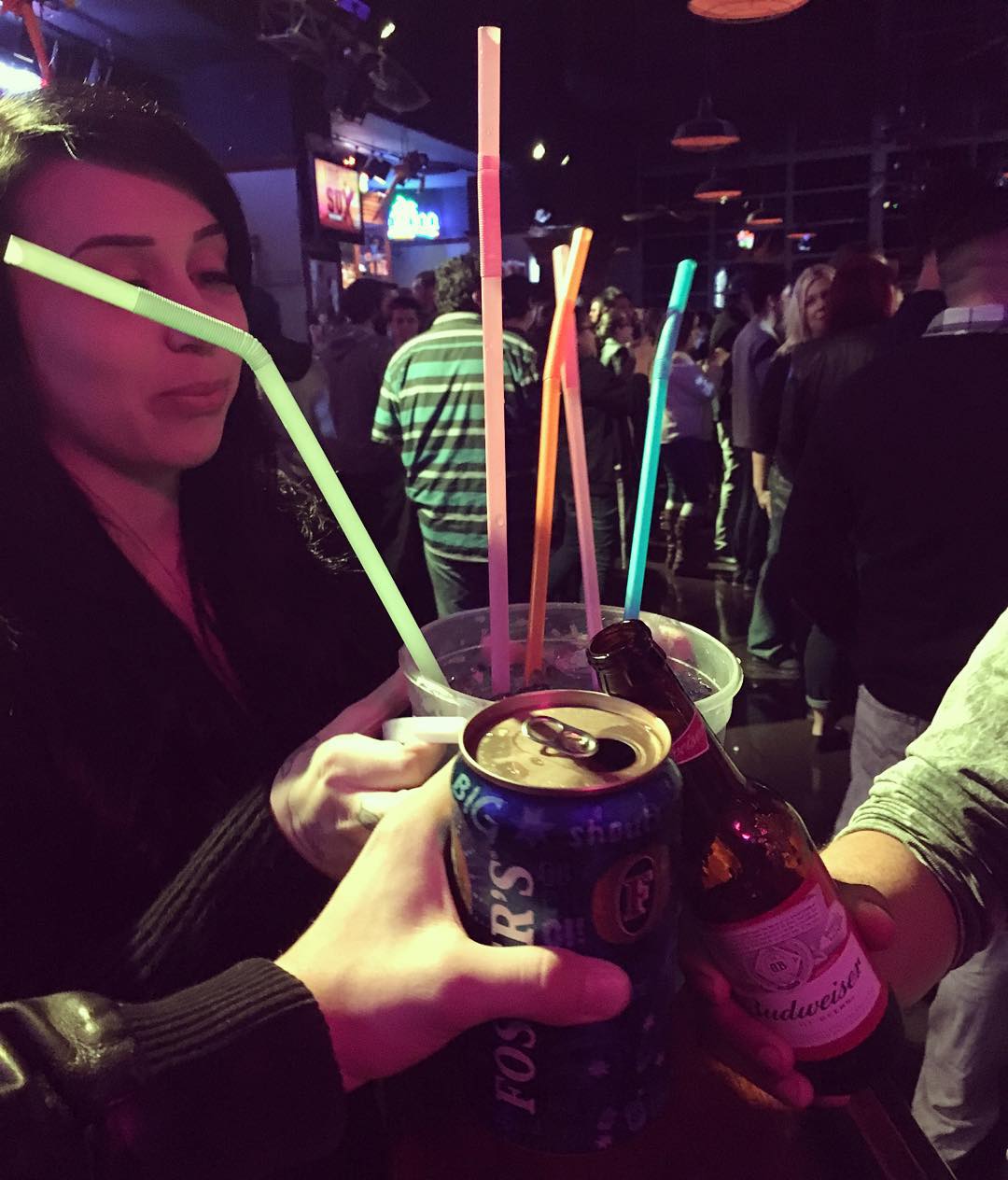In this vibrant, dimly-lit nightclub scene, the dark background is subtly brightened by dimmed, orange ceiling lights that curve towards the windows, hinting at the lively ambiance of the night. The club is bustling with casually dressed men and women scattered throughout, engaging in conversations and revelry. Dominating the foreground is a young white woman with dark hair and meticulously made-up eyebrows, wearing a long-sleeved black sweater. She holds an enormous drink tub adorned with five colorful straws in shades of light green, pink, orange, and teal. Toasting with her are two other individuals: one to her left, clad in a black sleeve featuring a gold pattern, raises a blue Foster's beer can, while the other to her right, in a green shirt with pushed-up sleeves, lifts a Budweiser bottle. They are all joining in a celebratory cheer, their drinks converging in the center of the frame, capturing a moment of shared excitement and camaraderie in this bustling nighttime locale.